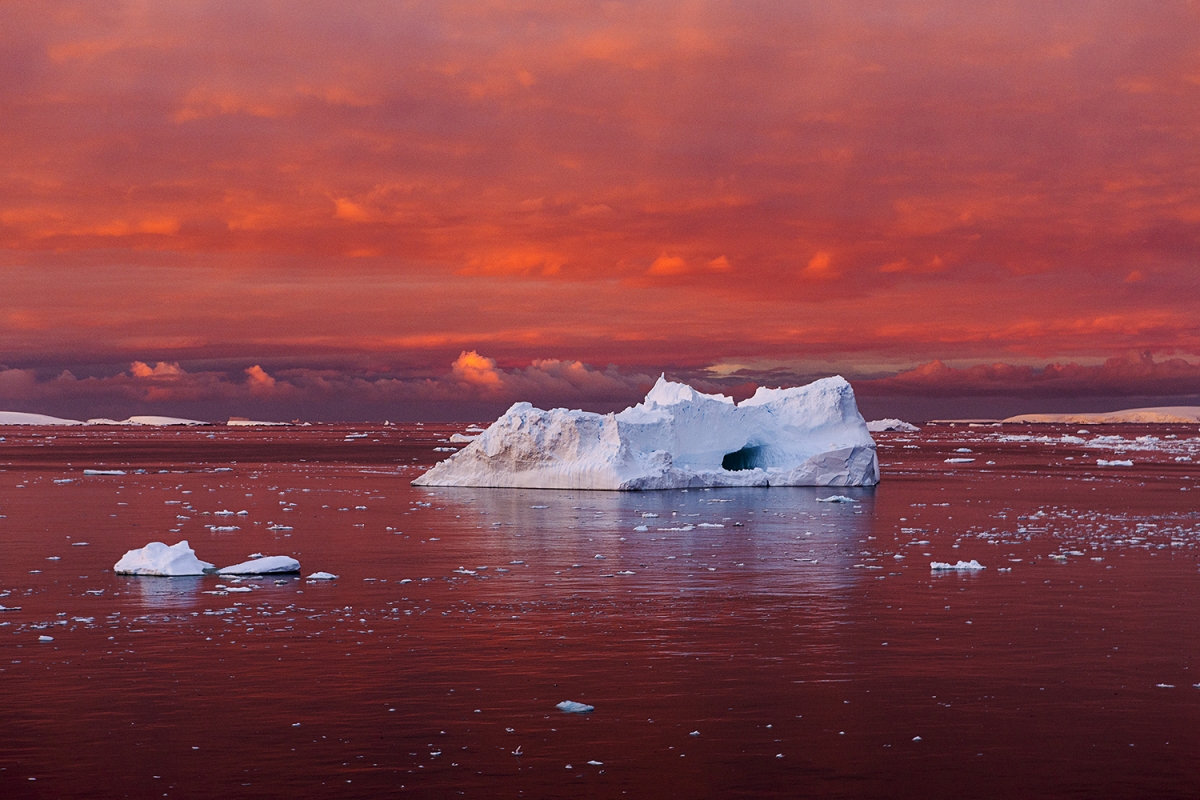In this stunning image captured during either sunrise or sunset in the far north, the sky is ablaze with shades of orange, pink, and purple, casting a spectacular glow over a vast, serene ice field. The sky is densely packed with mostly white clouds streaked with gray, all tinted by the sun’s radiant colors. In the distance, a majestic mountain range lies beneath a bank of clouds. The calm waters below mirror the vibrant sky, appearing red due to the reflection. Dominating the foreground is a large, flat iceberg with a cave-like indentation, rectangular in shape, surrounded by hundreds of smaller icebergs. These smaller ice chunks, scattered across the water, resemble floating snowballs or flat ice pieces. Additionally, a small patch of light brown land is visible on the right side of the image, further enriching the natural beauty captured in this breathtaking moment.